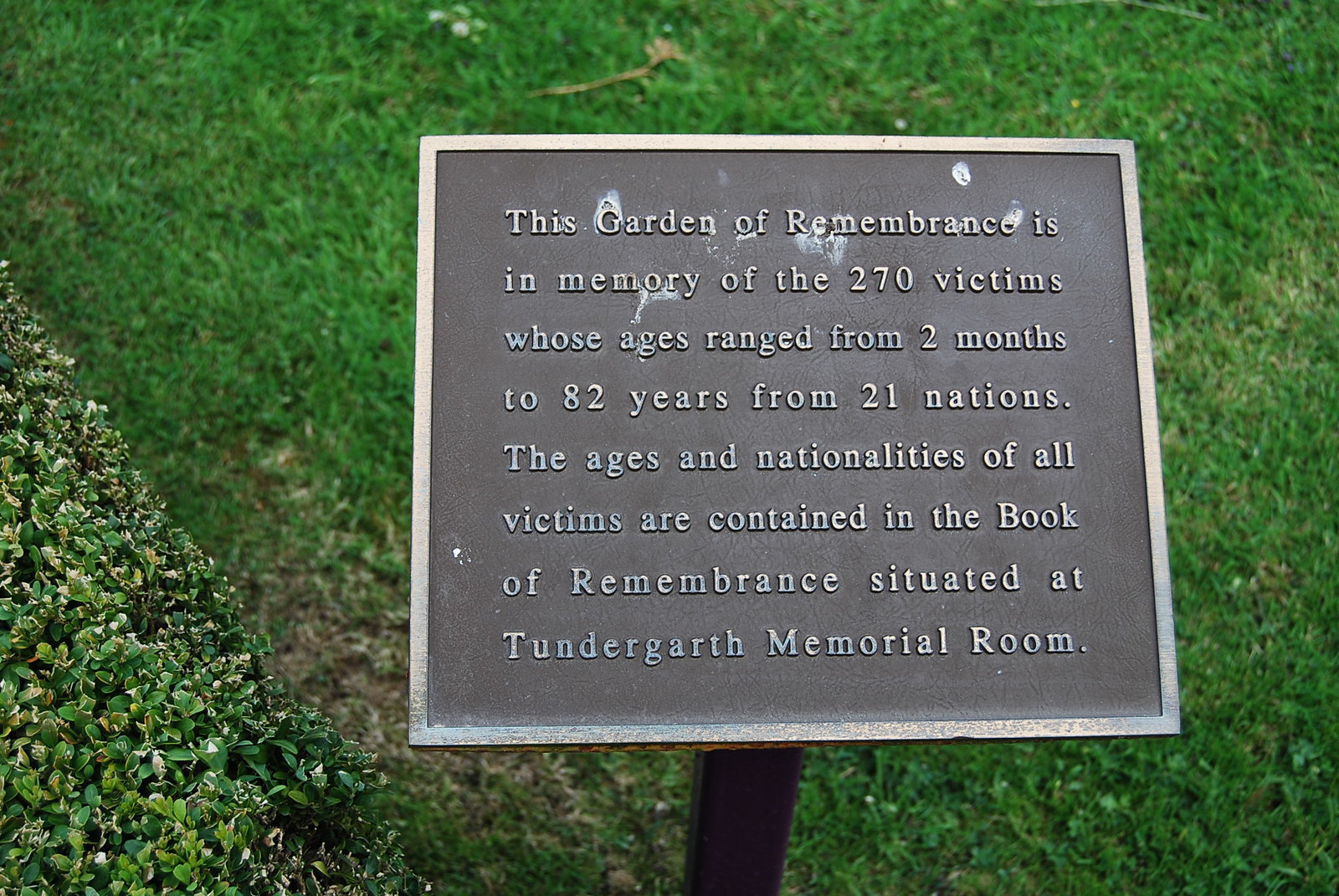In the center of this outdoor image, a black or dark gray metal plaque stands on a sturdy black pole amidst a well-manicured green field. The plaque, bordered in silver, bears raised silver text stating, "This garden of remembrance is in memory of the 270 victims whose ages ranged from two months to 82 years from 21 nations. The ages and nationalities of all victims are contained in the Book of Remembrance, situated at the Tundergarth Memorial Room." The grass surrounding the plaque is healthy and freshly trimmed, free of weeds, with no dead spots, and displays various shades of green. In the bottom left corner, there are neatly maintained bushes, possibly with small white flowers, adding to the serene atmosphere. A slight imperfection on the plaque, possibly bird droppings, hints at the natural setting, suggesting a historical or memorial garden, captured in the bright daylight.